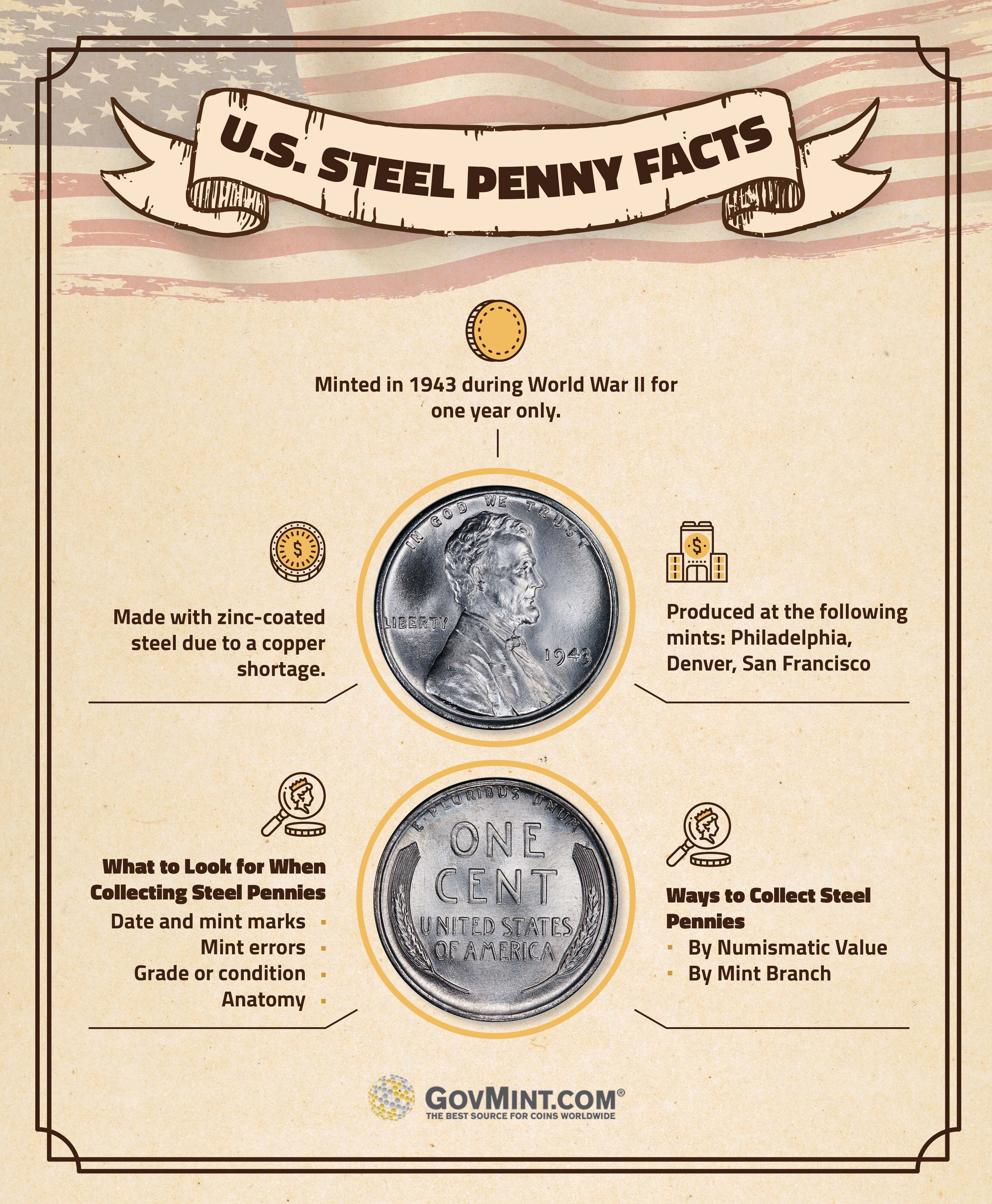The poster features an infographic with a tan paper-like background, showcasing detailed information about the U.S. Steel Penny. At the very top, there is an American flag, under which a bold banner reads "U.S. Steel Penny Facts." Below this, an illustration of a yellow coin is accompanied by the text "minted in 1943 during World War II for one year only."

The infographic is divided into sections. The first section illustrates the front (heads) and back (tails) sides of the steel penny. The heads side features an image of Abraham Lincoln in profile, with "Liberty" inscribed on it. The tails side shows "One Cent" and a depiction of two laurel leaves. Additional text around these images provides important context such as "made with zinc-coated steel due to a copper shortage" and notes that it was produced at the mints in Philadelphia, Denver, and San Francisco.

The infographic also gives tips for collectors, highlighting aspects like important dates and mint marks, potential mint errors, overall condition, and the penny’s anatomy. It additionally suggests ways to collect steel pennies, either by numismatic value or by mint branch. At the bottom of the poster, the website GovMint.com is listed for further information.